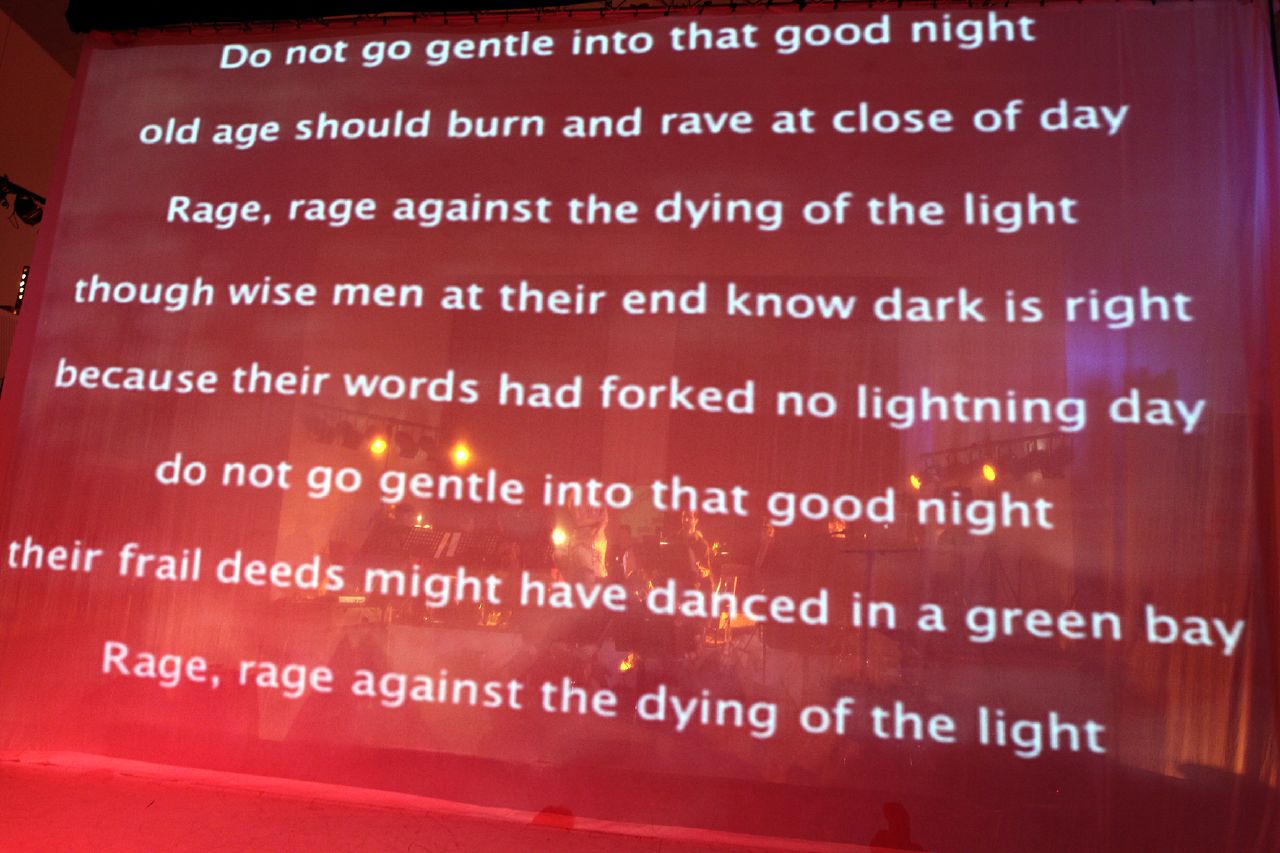The image depicts a translucent glass screen with a burgundy red backdrop and centered white text, likely part of a stage setup or teleprompter, reflecting various lights. Displayed on the screen is the renowned poem "Do Not Go Gentle into That Good Night". Each line of text is centered, starting with "Do not go gentle into that good night" and followed by "Old age should burn and rave at close of day," and "Rage, rage against the dying of the light." The poem continues with, "Though wise men at their end know dark is right" and "Because their words had forked no lightning day." The repetition of "Do not go gentle into that good night" and "Rage, rage against the dying of the light" emphasizes the fervent tone of the poem. The translucent quality of the screen allows the backdrop of stage lights and an orange wall to faintly appear, suggesting an event or performance setting.